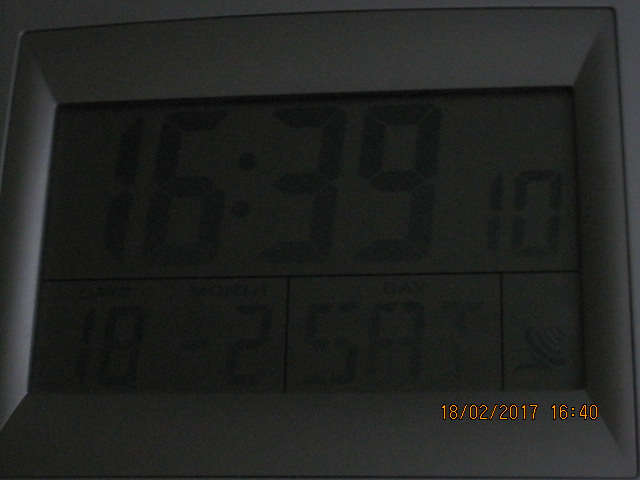This photograph captures an older-style digital clock with a grayscale face and very dark, almost unreadable numbers displaying the time as 16:39, indicative of 4:39 PM in a 24-hour format. The lower portion of the clock face appears to feature additional information, potentially including the date and air temperature, though these details are indistinct due to the image's low light conditions. The clock is encased in a silver-beveled frame. The photo itself has a visible watermark date of 18-02-2017, conforming to the European date format, which corresponds closely with the time shown on the clock. The overall darkness of the image makes it challenging to discern finer details, suggesting it may have been an original printed photograph.